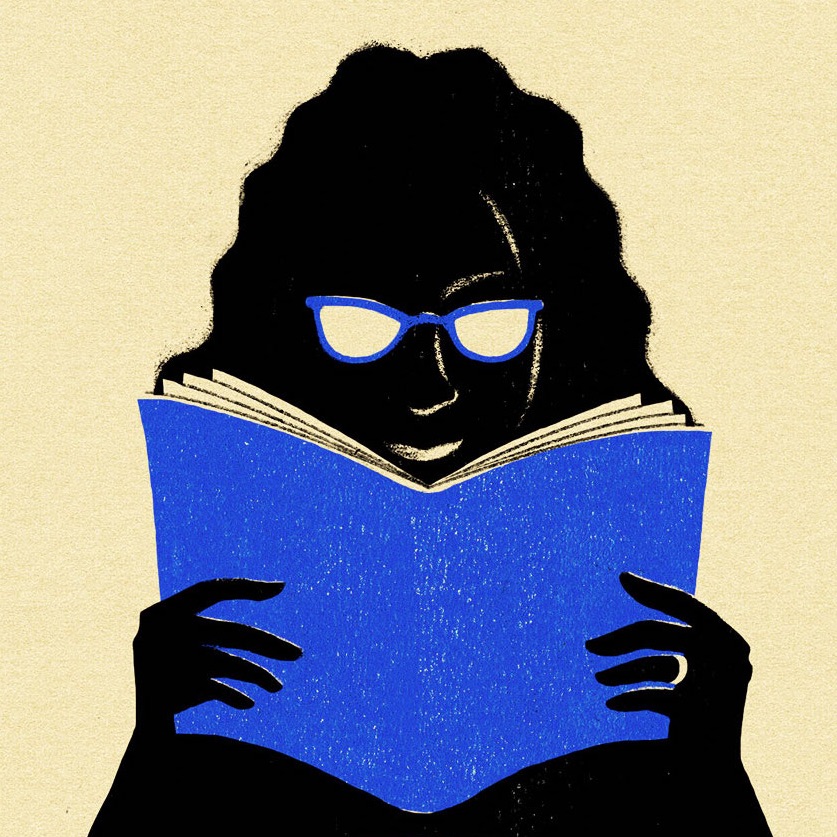This artwork appears to be a detailed block print or painting on a textured beige or recycled paper background. The central figure is the black silhouette of a woman from the chest up. She has distinct features highlighted with white line work, including her right cheek, nose, and a smiling mouth. These accents might be brush strokes or negative space details. The woman is holding an open blue book with white pages close to her face, and her left hand prominently displays a wedding ring on her ring finger. Her blue-rimmed glasses match the color of the book, with lenses that appear white, possibly reflecting light. The image exudes a sense of peaceful engrossment in reading, and it could be aptly used as a logo for a library or literary event. The minimalistic yet evocative design provides a serene and contemplative mood.